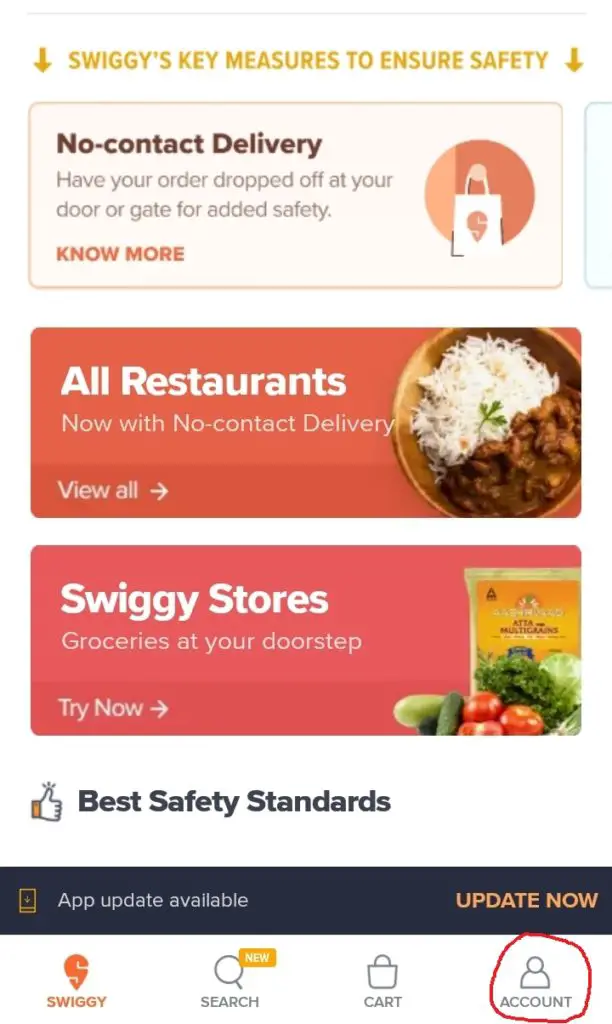The image depicts a detailed promotional update from Swiggy, highlighting their commitment to safety through "No Contact Delivery." For added security, your order can be left at your door or gate, minimizing physical interaction. The image also indicates that all partnered restaurants now offer this no-contact service. Additionally, viewers are encouraged to explore Swiggy Stores for groceries conveniently delivered to their doorstep. There is a prompt to update the Swiggy app to access the latest safety standards. The user interface shows options for Search, Cart, and Account, with a red circle emphasizing the Account section. In the visual foreground, there is a plate of rice and meat, symbolizing meal deliveries, alongside a shopping bag filled with fresh cucumbers, tomatoes, and broccoli, representing grocery deliveries.